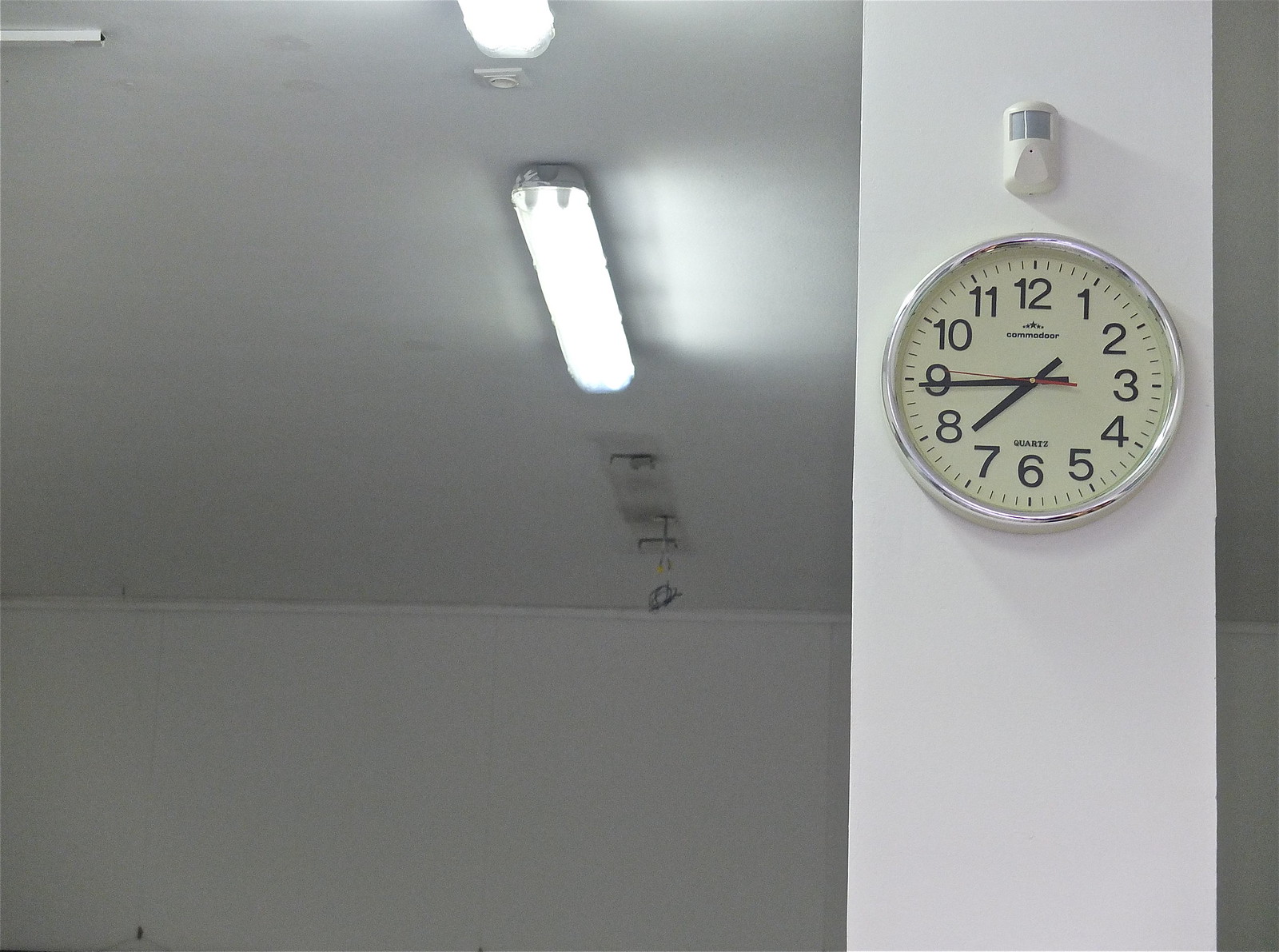This is a detailed photograph of a room with white walls and ceiling. On the right side of the room, there is a relatively skinny, rectangular white pillar taking up about one-fourth of the picture. Mounted on this pillar is a round clock with a shiny silver outer edge and an off-white, beige face. The clock features large black numbers, small black minute hash marks, and thicker black hour hash marks at each numbered position. It has two black rectangular hands for the hours and minutes, and a thin red rectangular hand for the seconds. The hour hand points just before 8, and the minute hand is almost at 9, indicating a time of approximately 7:45. Above the clock, there is a rectangular emergency light with two sensors. Additionally, the ceiling features a line of fluorescent lights; three are visible in the image, though the furthest one is missing its bulbs. There is also a small intercom with a grated front above the clock on the pillar.